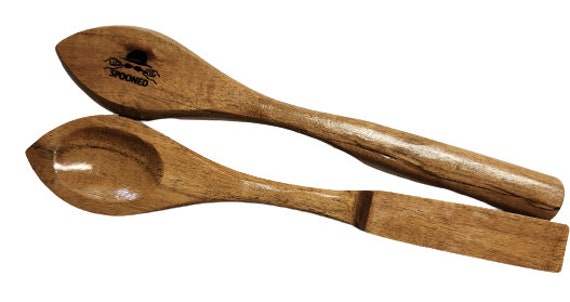The image features two wooden spoons, set against a white background. The bottom spoon is displayed with its concave, elliptical head facing up, revealing a well-worn, grooved surface that reflects light slightly, suggesting it is polished. The handle of this spoon is flat and rectangular, ending in a pointed tip that resembles the shape of a pitted avocado. The wood grain is visible, characterized by its darker hue, and the overall design suggests a primitive, handmade quality.

Above this, the second spoon is shown in reverse, with the back of its head facing the viewer. This spoon also has a pointed tip at its head, but features a more rounded handle compared to its counterpart. Burnt into the back of this spoon is a black logo resembling a hat and sunglasses, accompanied by the word “spooned” in black text, indicating it may be a product of a specific company rather than an antique. The spoons appear sturdy and robust, crafted from dark, grainy wood, reinforcing their handcrafted aesthetic.